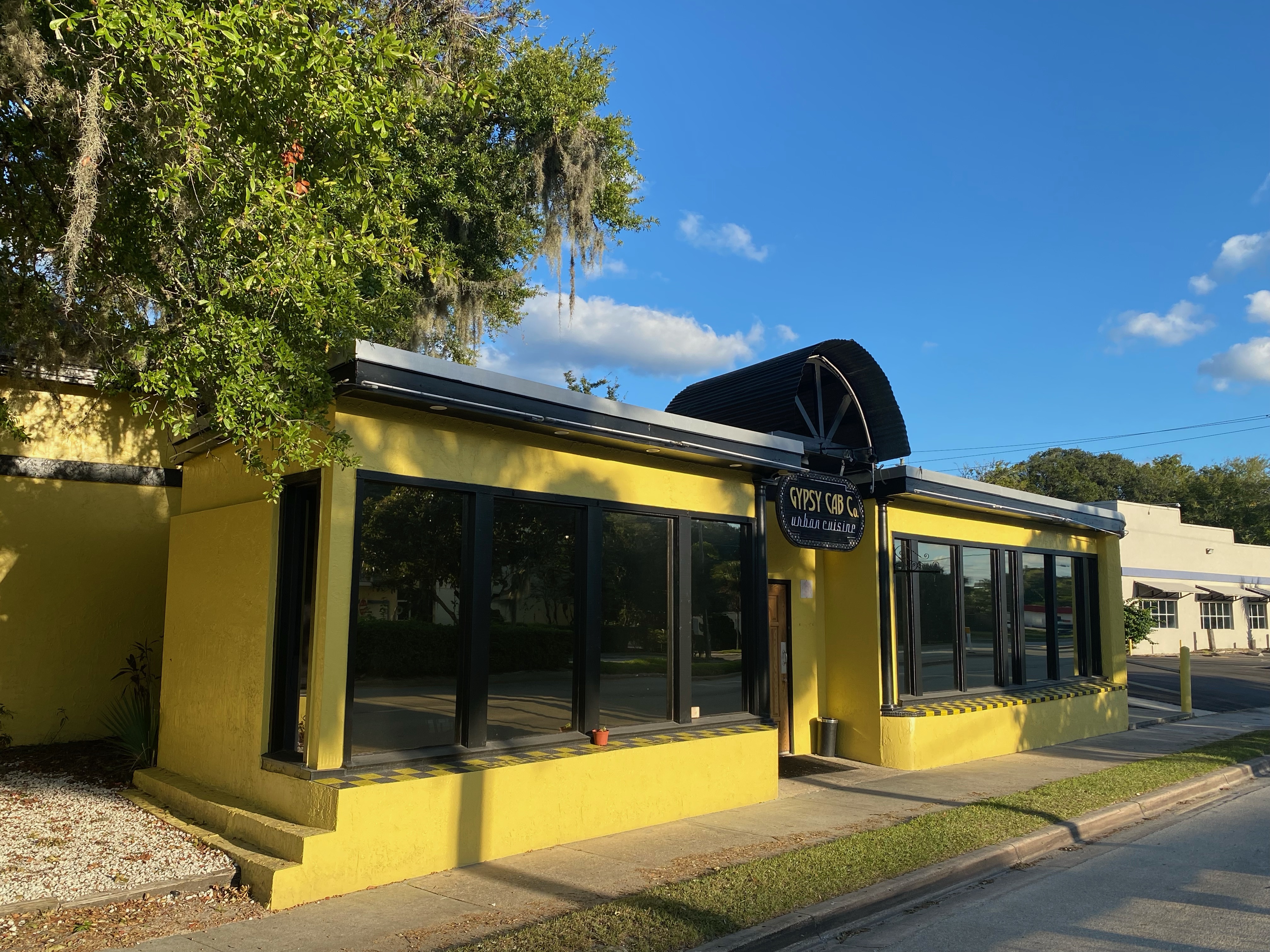The photograph captures a daytime view of the exterior of a business named "Gypsy Cab Company." This establishment is housed in a wide, rectangular building painted a vibrant yellow. Above the doorway, a placard with the business name is prominently displayed, accompanied by some smaller, harder-to-read white text underneath. The facade features large, tinted windows flanking the entrance on both sides, creating a balanced and welcoming aesthetic.

A significant architectural detail is the large overhang in front of the building, equipped with recessed lighting along the top, which likely illuminates the entrance during evening hours. The entrance itself is highlighted by a curved archway, adding a touch of elegance to the structure.

In front of the business, a narrow crosswalk spans a grass border that separates the sidewalk from the curb. In the background, another beige-colored building with multiple windows adorned with awnings can be seen. The sky is a clear blue with scattered white clouds, adding to the photograph's vibrancy. Additionally, the branches of a tree, likely situated right next to the building, overhang slightly, adding a hint of greenery to the scene.